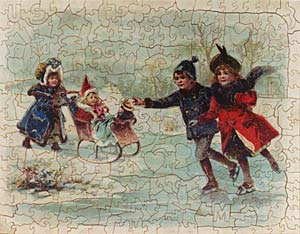In a quaint and nostalgic winter scene depicted in a small square image reminiscent of a puzzle piece from decades past, two young children, a boy in a blue jacket and a girl in a red coat with a flowing scarf, skate hand-in-hand on a frozen pond situated on the right side of the frame. On the left, a woman in a heavy coat and hat is seen pushing a stroller, strikingly styled like Santa's sleigh with runners instead of wheels. The stroller appears to cradle a bundled-up baby donning a Santa hat and possibly accompanied by a small dog. The serene winter setting is painted in an array of colors including reds, blues, whites, blacks, grays, browns, and light greens, blending harmoniously with the icy blue expanse and white-edged landscape under a matching blue sky.